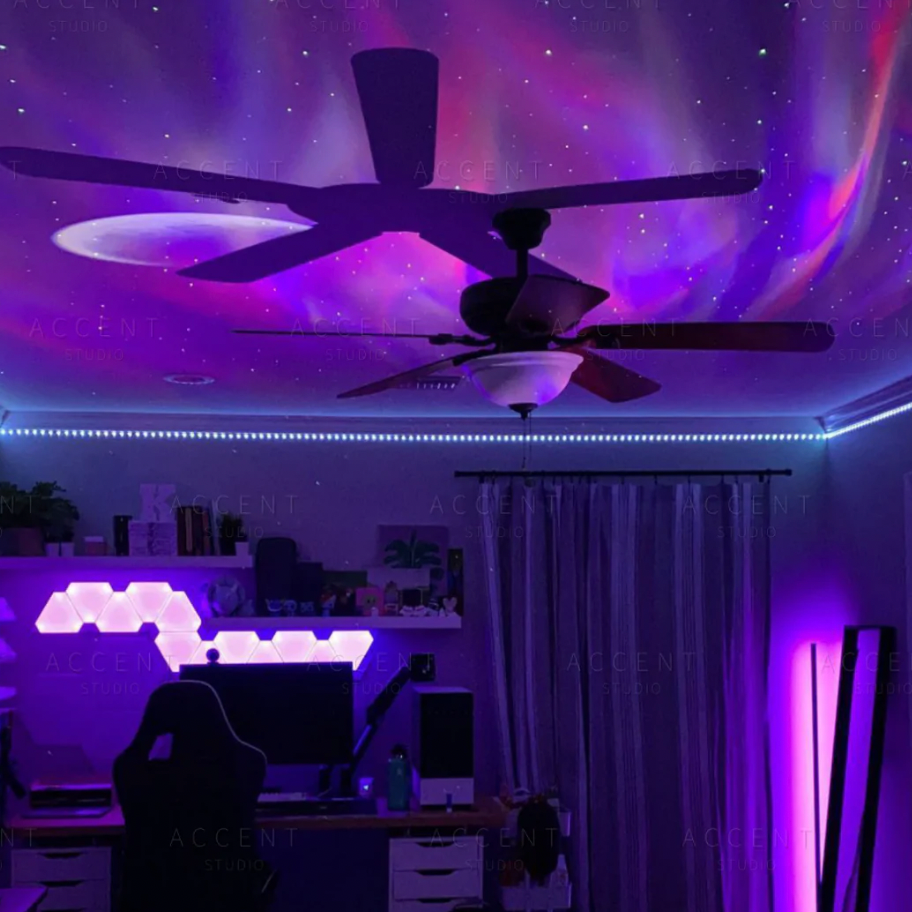This photograph, taken indoors at night, reveals a bedroom bathed in a captivating purple glow, suggestive of black light illumination. The square-shaped image, about five to six inches in dimensions, centers around the partition between the ceiling and the sidewall. The ceiling, adorned in purple and pink tones and adorned with dot-like stars and a painted or projected moon, features a central ceiling fan with a white lampshade and five brown wooden blades. The fan's shadow extends to the upper left of the ceiling.

To the right of the image, blue beaded LED lights run along the top of the back and right walls, leading down to closed curtains. Below, a computer desk with a computer and a chair sits against the left wall, flanked by floating shelves. Triangular LED lights connect above the computer but below the shelves, contributing to the space-themed decor. The backdrop includes a mirror leaning up against the wall and various glowing shapes and graphics in white. A watermark across the image reads "Accent Studio."